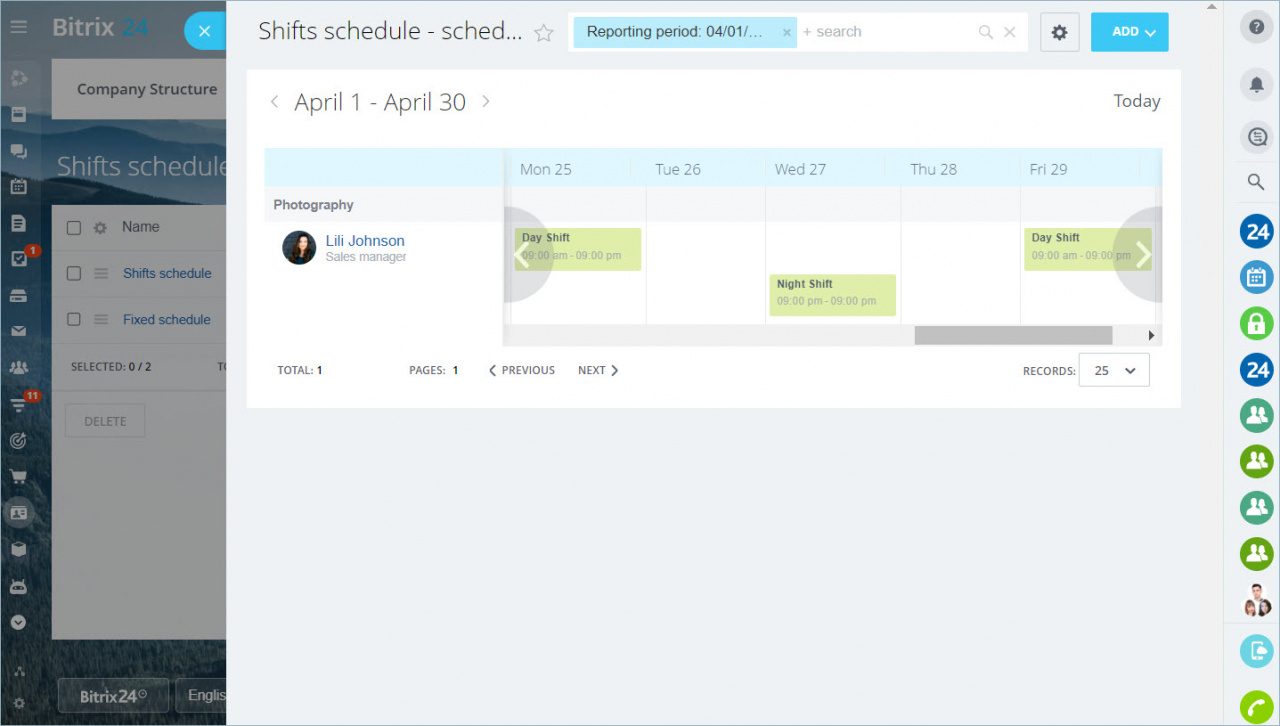This image is a screenshot captured from a Bitrix24 software application, typically used by private companies for various organizational needs. The screenshot prominently features a pop-out window displaying a detailed daily calendar-style shift schedule for Lily Johnson, the sales manager in the photography department, for the period from April 1st to April 30th. The background has a translucent overlay, through which the Bitrix24 logo is discernible. On the left side of the screen, there is a vertical list of small icons, among which the "Company Structure" button can be seen. This button, when activated, displays a table listing both shift schedules and fixed schedules for the company's employees. The pop-out window in focus elaborates on Lily Johnson’s work shifts, clearly indicating whether she is assigned to day shifts or night shifts on specific dates within the given month.